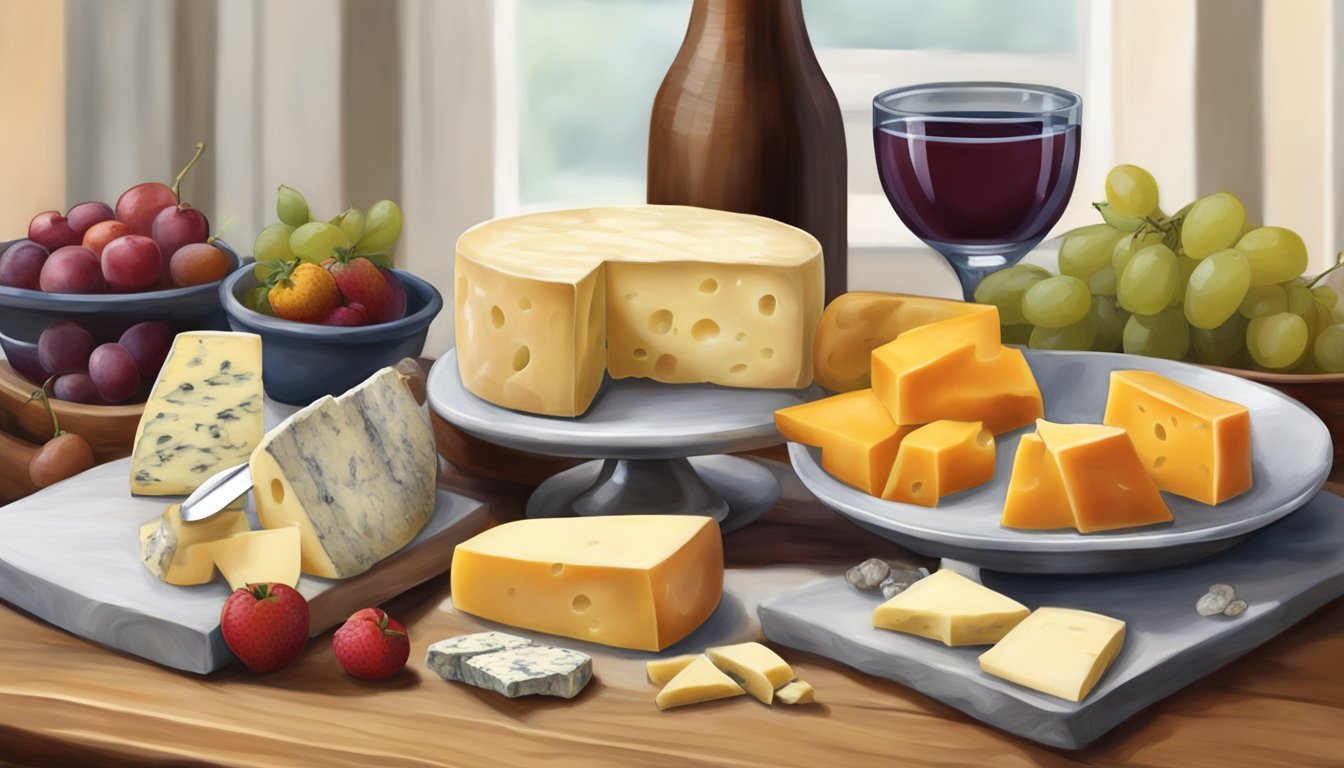This image is a detailed painting or digital illustration of a wooden table set up for a wine and cheese hour, bathed in the sunny light from a window in the background. Central to the composition are various cheeses displayed on both blue and gray plates as well as marble trays. Visible cheeses include blue cheese, cheddar, and a large wheel of pale yellow Swiss cheese with characteristic holes and a triangular chunk cut out. There's also an orange-hued cheese and a marbled cheese streaked with blue. Bowls of fruit, including purple and green grapes, apricots, plums, and strawberries, are distributed across the table. In the background, there is a tall brown bottle of wine, and next to it, a large wine glass filled with red wine. The entire scene is rich with colors—yellows, browns, purples, and greens—evoking a warm, inviting atmosphere perfect for entertaining guests.